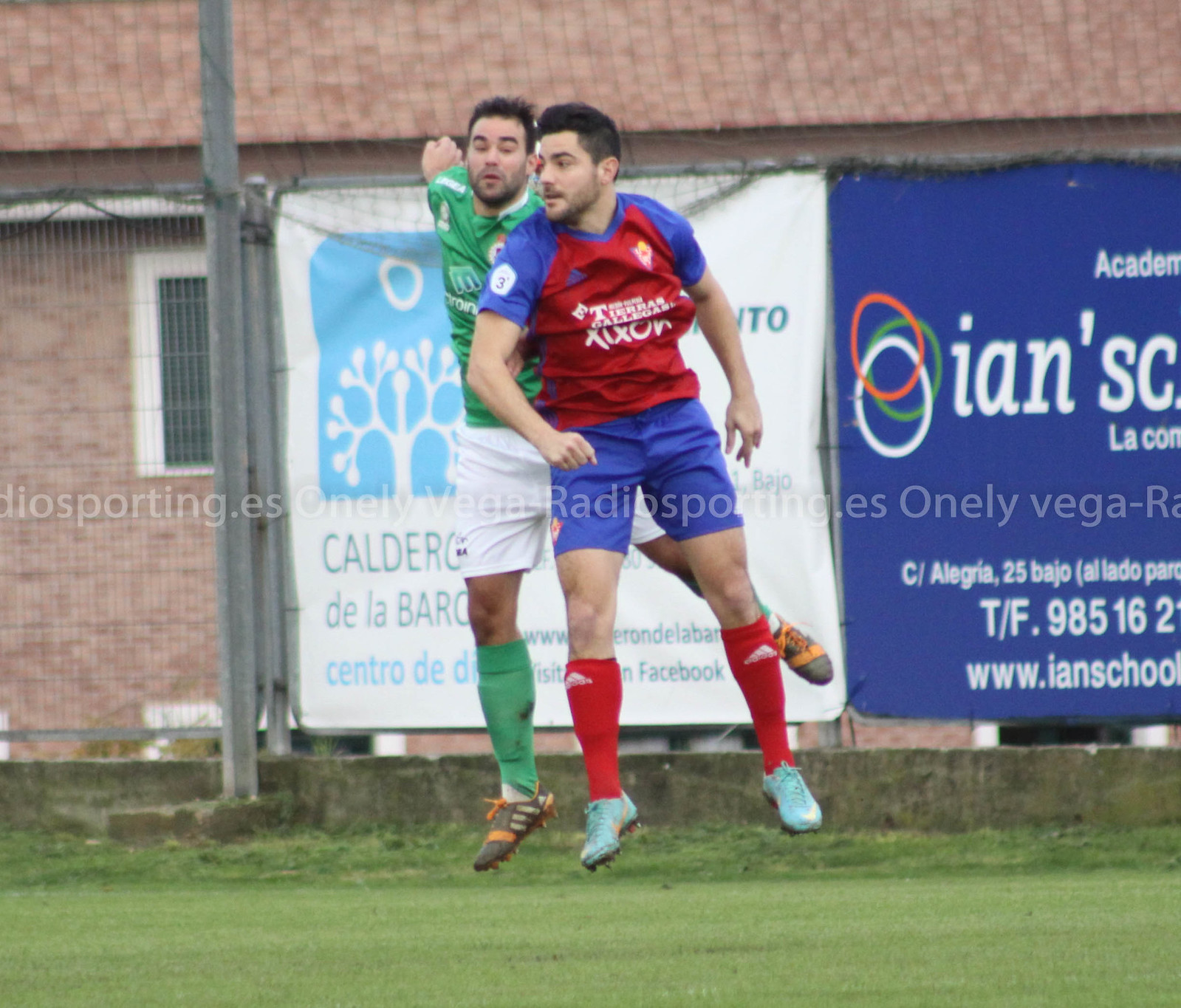This is a large, square outdoor photograph capturing two soccer players mid-action, seemingly colliding in midair, possibly after jumping while going after a ball that is off-frame. The detailed uniforms reveal one player in a red and blue ensemble with long red socks up to his knees and turquoise cleats, while the other player sports a green shirt, white shorts, green knee-high socks, and gray and orange cleats. Below them, the green field is visible. The backdrop showcases a series of advertisements, including audiosporting.es and onelyvegasradiosporting.es. The backdrop is adorned with vibrant colors—blue, white, orange, and green—and features various graphics, including a tree symbol and additional white writing with a telephone number and a website. To the left of the backdrop is more fencing, and peeking above it, the roof of another structure is visible. The dynamic moment captures the high energy and intensity of the match.